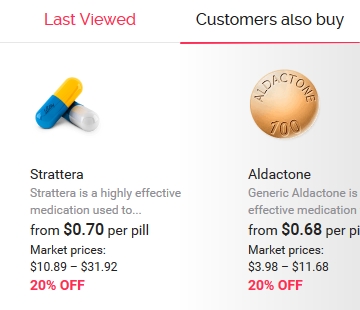The image displays a segment of a laptop screen featuring a web page with a white background. At the top, typical elements such as the time, date, Wi-Fi strength, and battery status are notably absent. Below this blank space, there is a search interface with a top bar showing sections labeled "Last Viewed" in red and "Customers Also Buy" in black, the latter highlighted by a red underline.

Under the "Last Viewed" section, the medication "Stratera" is showcased. The product image includes two types of capsules: one blue and gold, and another white and gold. The description indicates that Stratera is a highly effective medication, though the text is truncated and unreadable. Pricing details show it costs from 70 cents per pill, with a market price ranging from $10.89 to $31.92, and a current discount offering 20% off.

To the right of Stratera, another medication, "Alcaton," is displayed in tablet form. The description mentions it as a generic version, though specifics are partially obscured, referring to it as an effective medication. Its pricing is listed at 68 cents per pill, with a market price between $3.98 and $11.68, also featuring a 20% discount.

The overall impression is of an online pharmaceutical retail platform where discounted medications are being prominently advertised.